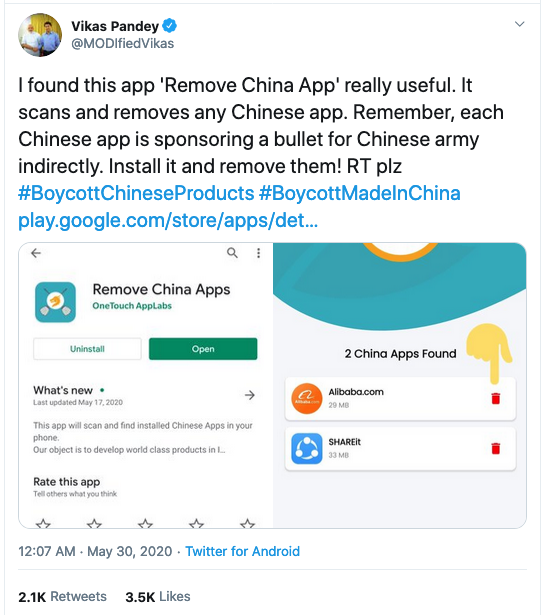**Caption:**

This image is a detailed screenshot of a tweet by Vikas Pandey, a verified Twitter user, as indicated by the blue check mark next to his name in bold. His profile picture features two men, one in a white shirt and the other in a blue shirt. His Twitter handle is @ModifiedVikas.

The tweet, posted on May 30th, 2020, at 12:00 AM from Twitter for Android, highlights Vikas Pandey's endorsement of an app called "Remove China Apps" by OneTouch Labs. He commends the app for its ability to scan and remove Chinese applications, advocating its use with a rather strong statement about the implications of using Chinese apps. The tweet ends with a call to action for retweets and includes hashtags #boycottChineseproducts and #boycottMadeinChina, along with a link to the app on the Google Play Store.

The image also includes screenshots of the "Remove China Apps" interface, showing that it has detected two Chinese apps on Pandey's device. His tweet has garnered significant interaction, with 2.1 thousand retweets and 3.5 thousand likes.